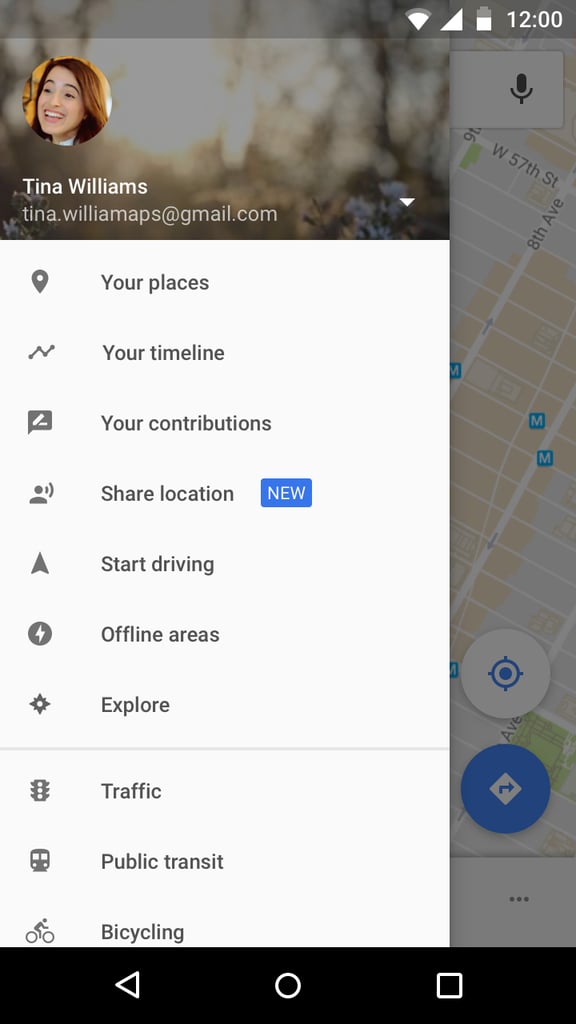This vertical image appears to be a screenshot from a smartphone taken during the golden hour, as the warm sunlight filters through the trees in a wooded area, creating a blurred, glowing background. On the left-hand side, there is a small circular profile picture of a person with the name "Tina Williams" written in white text underneath, followed by her email "Tina.WilliamAPS@gmail.com." 

In the upper-right corner, there are various status icons, including a triangle, Wi-Fi signal, battery life, and the time displayed as 12:00. Below these icons, there is a small black microphone icon on a white box. 

On the left-hand side of the screen, there is a vertical, rectangular white box displaying a list with icons preceding each entry. The list includes: "Your places," "Your timeline," "Your contributions," "Share location" with a blue box beside it labeled "NEW" in white uppercase letters, "Start driving," "Offline areas," and "Explore." A thin gray line separates this list from the next section, which features options for "Traffic," "Public transit," and "Bicycling." 

At the bottom of the screen, a black strip houses three navigation icons: a white triangle pointing left, a circle in the center, and a square on the right. 

This image is detailed and structured, indicative of a user interface from a mapping or navigation application.